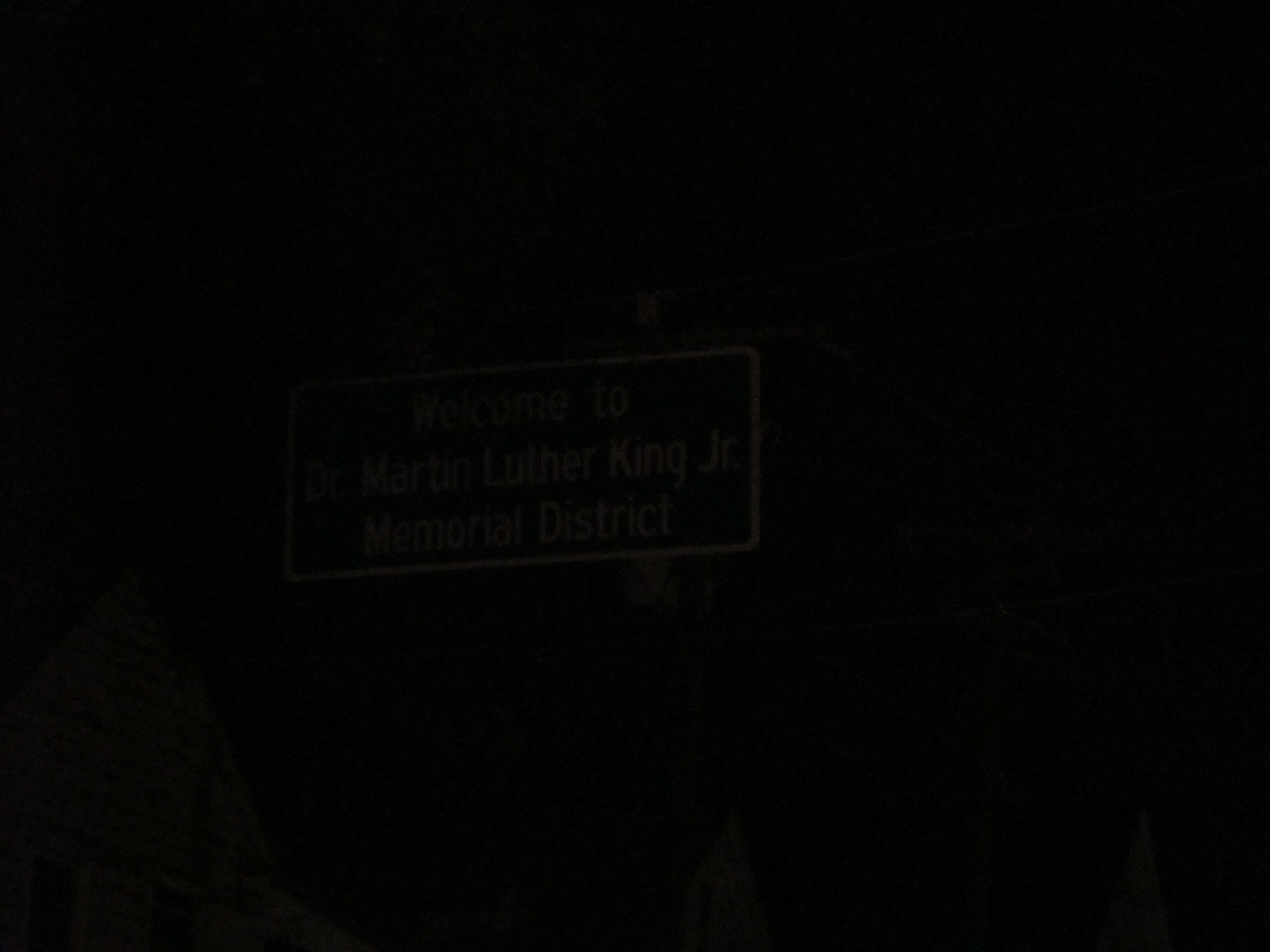The image is predominantly dark, either intentionally or due to severe underexposure, making it difficult to discern most of its contents. At the center of the near-black frame, a sign is barely visible. The sign features a distinct white outline, creating a faint but noticeable contrast against the dark background. The sign resembles a road sign and contains text in white font. The text is distributed over three lines: "Welcome to" on the first line, "Dr. Martin Luther King Jr." on the second line, and "Memorial District" on the third line. Despite the image's darkness, the white outline and font allow for the sign's message to be partially discernible within the obscure setting.